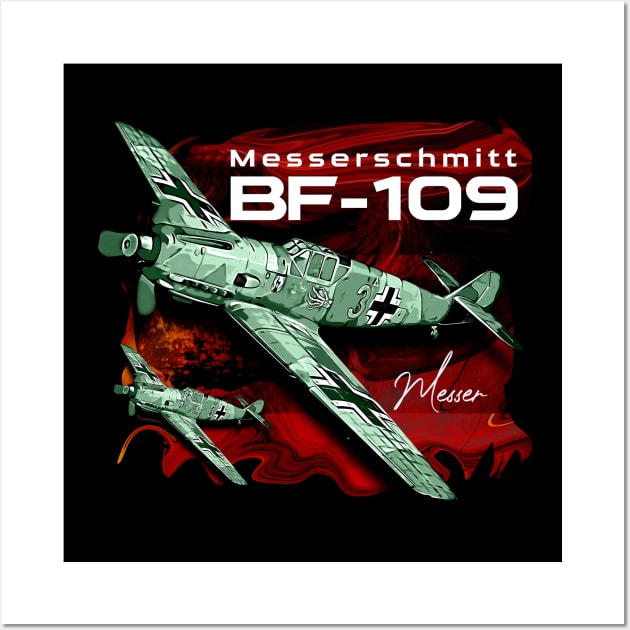The image is a detailed cartoon-style illustration of a World War II-era German Messerschmitt BF-109. The drawing features a prominent plane in the center, depicted in a green and gray color scheme with distinctive black crosses bordered in white on the wings and tail. This central plane also sports a shark-like face design near its front, adding a touch of character, and has the number three painted on its side near the cockpit. The illustration includes a smaller rendition of the same plane, positioned slightly lower and to the left of the central image. Both planes showcase clear details such as front and side windows, propellers, and tail sections. The background is swirled with black and red hues, and the entire scene is framed by a white border. The top of the image bears the text "Messerschmitt BF-109" in white letters over the red portion of the background. In the bottom right-hand corner, the artist’s signature "Messer" is elegantly written in white cursive.